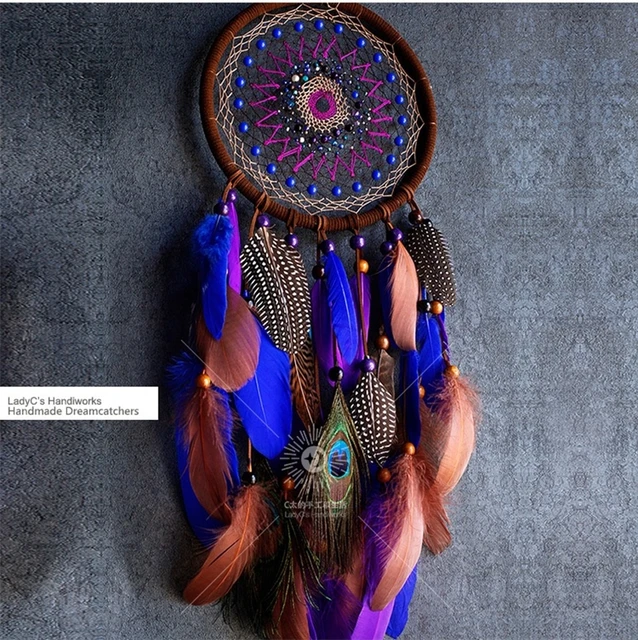The image showcases a beautifully handcrafted dreamcatcher, typically recognized as a piece of Native American art. The central hoop, crafted from brown wood-like material, is intricately woven with multiple layers of string in a detailed pattern. The outermost layer utilizes white string interspersed with blue beads, followed by black and purple string adorned with multicolored beads. The innermost layers feature alternating white and purple string, enveloping the design in a harmonious color scheme.

Suspended from the hoop are seven rows of elegant feathers, totaling 10 to 15, in an array of colors including blue, purple, light orange, and rust, alongside notable brown and white-spotted feathers. Among these, a distinctive peacock feather adds a touch of vibrancy. The dreamcatcher is positioned against a bluish-gray felt backdrop, enhancing the intricate details of the web-like pattern and the delicate features of the hanging feathers.

Beside the dreamcatcher, there is a sign that reads "Lady C's Handiworks Handmade Dreamcatchers," attributing the creation to an artisanal source. This intricate piece, rich in color and craftsmanship, embodies traditional elements while showcasing a modern palette and design.